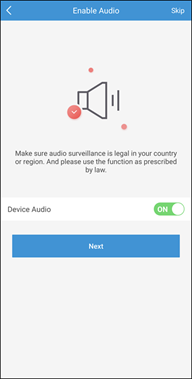This image appears to be a cell phone screenshot displaying an audio permissions interface. At the top center of the screen, white text reads "Enable Audio." In the top right-hand corner, there's a "Skip" button, while the top left-hand corner features a back button symbolized by a leftward-pointing arrow.

Dominating the center of the image is a small, black-outlined speaker icon. Underneath, a message warns users: "Make sure audio surveillance is legal in your country or region. Also, please use the function as prescribed by law." Following this text are options to turn the device audio on or off.

Toward the bottom of the screen, a prominent blue rectangular button with white text offers the next step with the word "Next" centered within it. The entire background of the interface is white, creating a clean and minimalistic appearance.

This screenshot evidently relates to a prompt for enabling audio permissions on a mobile device.